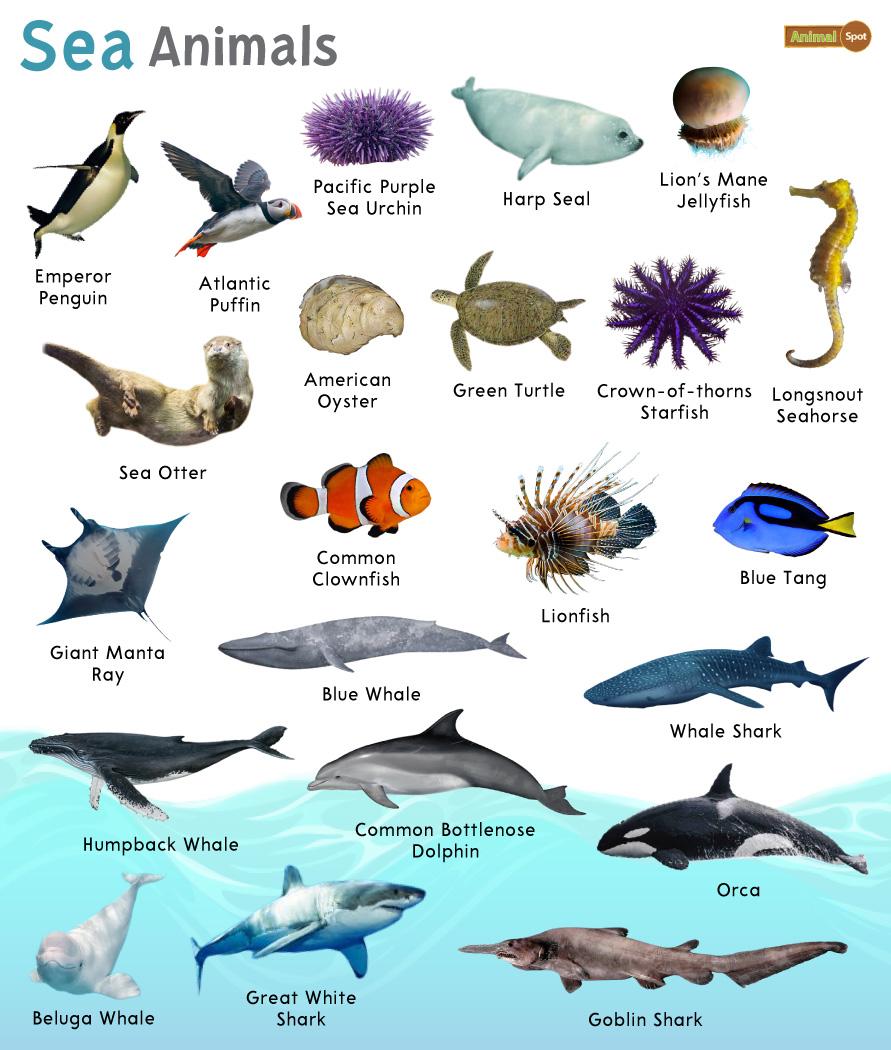The poster, titled "Sea Animals," features an intricate depiction of various marine creatures, with the word "Sea" in turquoise and "Animals" in gray. On the right-hand side, it reads "Animal Spot." The image is divided into five rows of labeled animals, with the bottom two rows shown underwater against a blue background. Starting from the top, the sequence includes: 

1. **Emperor Penguin** (black and white with an orange beak), **Atlantic Puffin**, **Pacific Purple Sea Urchin** (prickly), **Harp Seal** (gray), and **Lion's Mane Jellyfish** (tentacled).
  
2. **Sea Otter** (furry), **American Oyster** (textured), **Green Turtle** (shiny), **Crown of Thorns Starfish** (purple with distinctive tentacles), and **Long-Snout Seahorse** (notable for its elongated snout).

3. **Gray Manta Ray**, **Common Clownfish** (orange and white with black fin edges), **Lionfish** (with a mane-like appearance), and **Blue Tang** (neon blue and yellow-tailed).

4. **Humpback Whale** (black and white), **Blue Whale**, **Common Bottlenose Dolphin** (with a distinct fin), and **Whale Shark** (resembles a whale).

5. **Orca** (black and white), **Beluga Whale** (rounder, light gray, friendly face), **Great White Shark** (more gray and ominous), and **Goblin Shark** (dark gray, with a swordfish-like look).

The poster has a predominantly white background with about 25% of it resembling underwater scenes. The top right corner contains an unreadable logo.